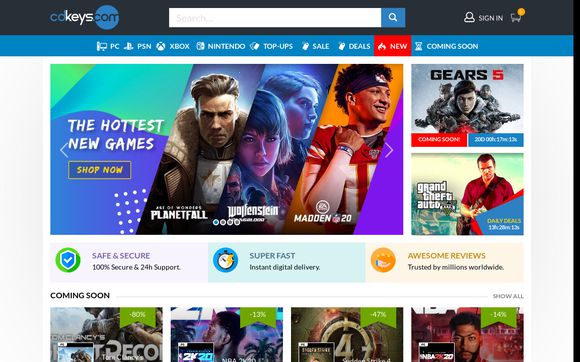A cropped screenshot of a browser displaying the cckeys.com homepage. At the top, the site’s logo is prominently visible beside a search bar featuring a blue square with a magnifying glass icon. Adjacent to these are options for "Sign In" and a shopping cart icon.

Directly below, a blue navigation banner displays various categories: PC, PSN, Xbox, Nintendo, Pop-ups, Sale, Deals, New, and Coming Soon. The "New" category is highlighted in red. Following this is the main page with a clean, white background. 

The top section showcases a large banner advertising "The New and Hottest Games," with a call-to-action button saying "Shop Now." This banner includes angled strips displaying game covers for *Planetfall*, *Wolfenstein*, and *Madden 20*. 

To the right of this banner, there are two stacked boxes highlighting more featured games: the top box promotes *Gears 5*, while the lower one features *Grand Theft Auto*.

In the center section, three informative boxes are presented: "Safe and Secure," "Super Fast," and "Awesome Reviews." At the bottom of the screenshot, the tops of four additional game images are visible, accompanied by the text "Coming Soon."